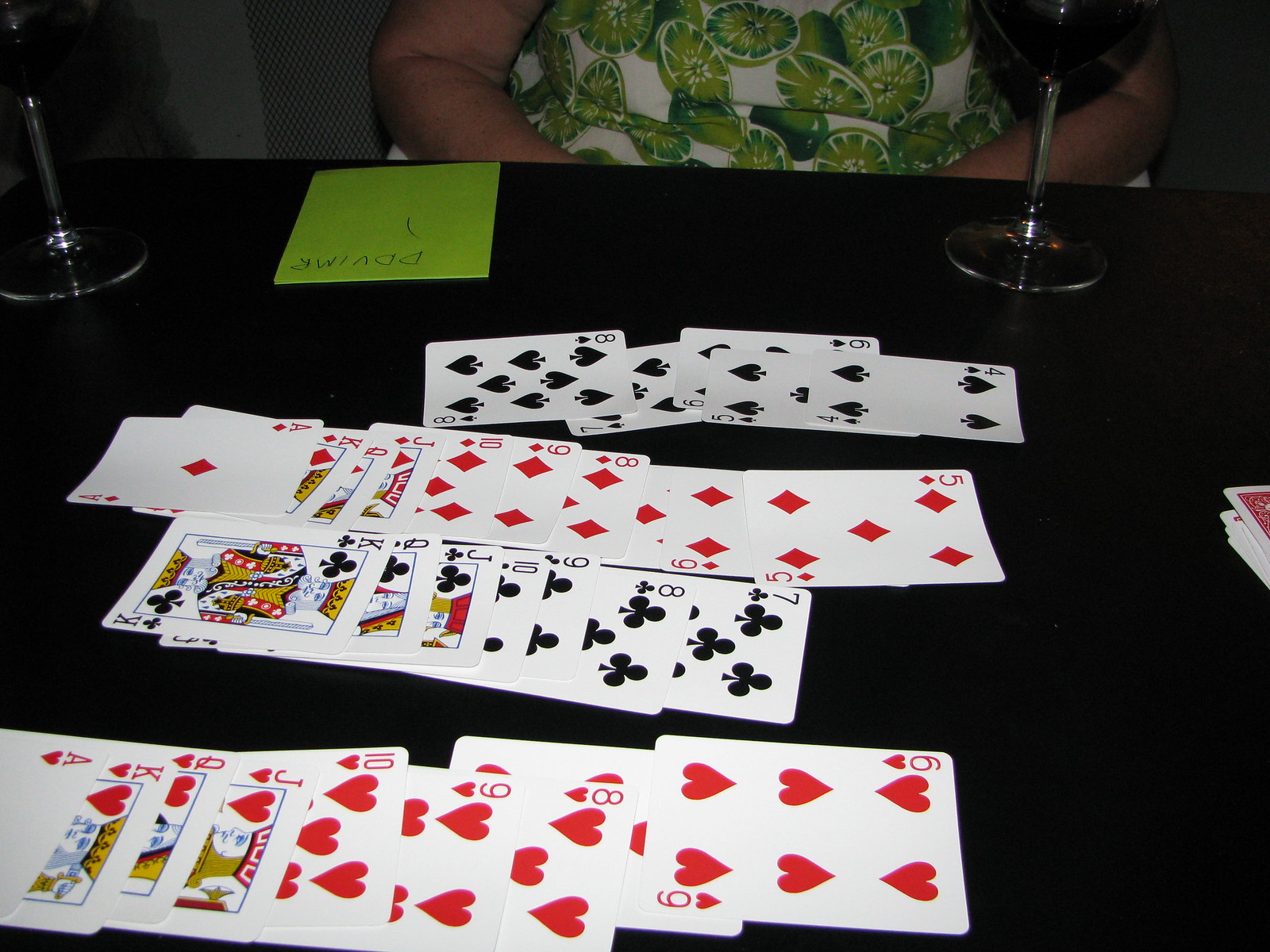A photograph captures a meticulously arranged card game on a sleek black table. At the bottom, there is a row of heart-suited cards neatly aligned: ace, king, queen, jack, ten, nine, eight, and six of hearts. Above them, another array showcases club-suited cards in a similar order: king, queen, jack, ten, nine, eight, and seven of clubs. In the next row, diamond-suited cards are displayed: ace, king, queen, jack, ten, nine, eight, six, and five of diamonds. Yet another row presents spade-suited cards: eight, seven, six, five, and four of spades.

Above the rows of cards, two half-filled wine glasses are placed on the table, suggesting a leisurely game night. A yellowish-green piece of paper with the text "D-D-V-I-M-R 1" lies nearby, possibly part of the game or a scorecard. At the very top of the image, a person is visible, clad in a distinctive white shirt adorned with green lime patterns, adding a playful and casual touch to the scene.